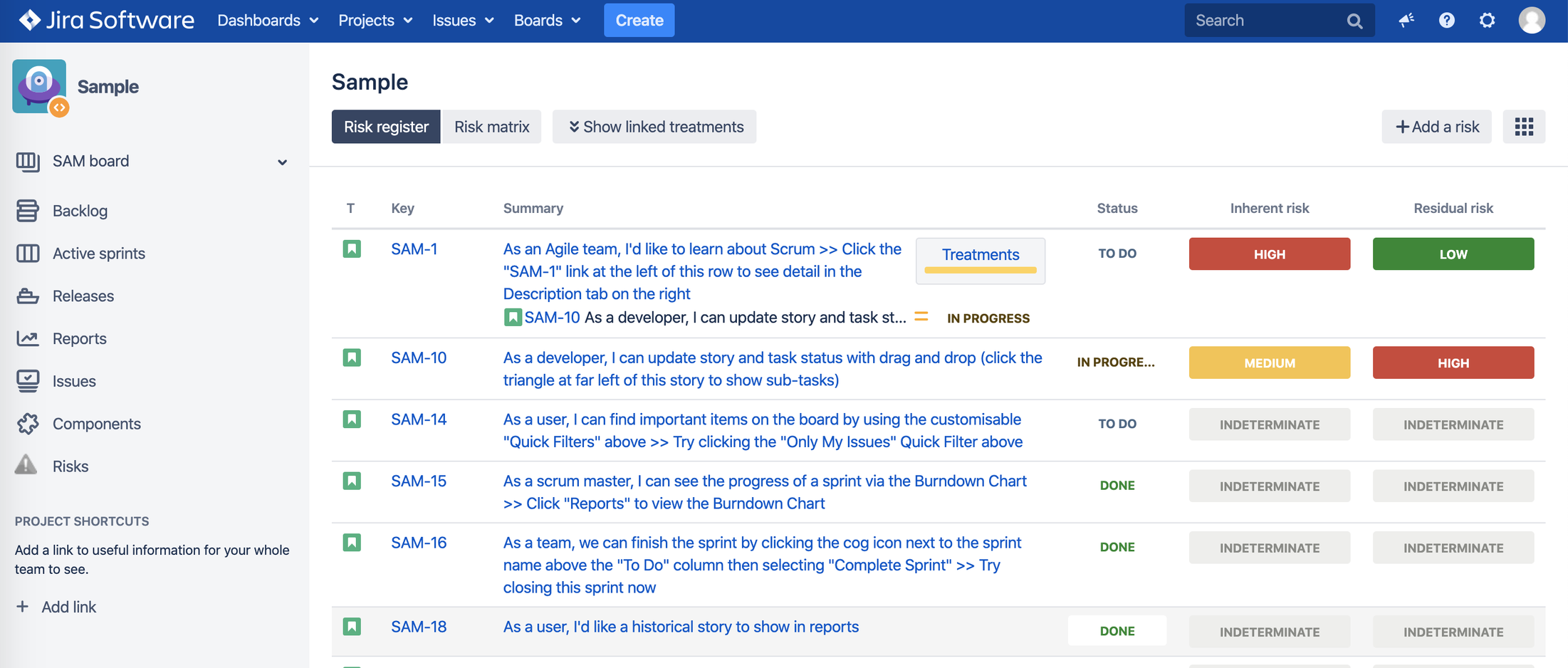This is a detailed screenshot of a JIRA software interface, showcasing various functionalities and sections. The navigation panel on the left side features multiple options such as 'Projects', 'Dashboards', 'Issues', 'Boards', 'Active Sprints', 'Releases', 'Reports', 'Components', 'Project Shortcuts', and an 'Add a Link' button. Within the 'Projects' section, there are entries like 'Sample' and 'Backlog'.

The main dashboard prominently displays a sample 'Risk Register' with several columns. The columns are labeled 'T', 'Key', 'Summary', 'Status', 'Inherent Risk', and 'Gradient Risk'. For instance, the 'Key' column lists items with designations like 'SAM-1', followed by their corresponding summaries. The 'Status' column indicates the current state of each item, shifting between statuses such as 'To Do', 'In Progress', and 'Done'. Users can rank these risks to prioritize tasks based on their importance, referenced by the 'Key' column identifiers.

The interface also highlights a color-coded system with red, yellow, and green buttons, presumably used to signify different states or priority levels of tasks and risks.